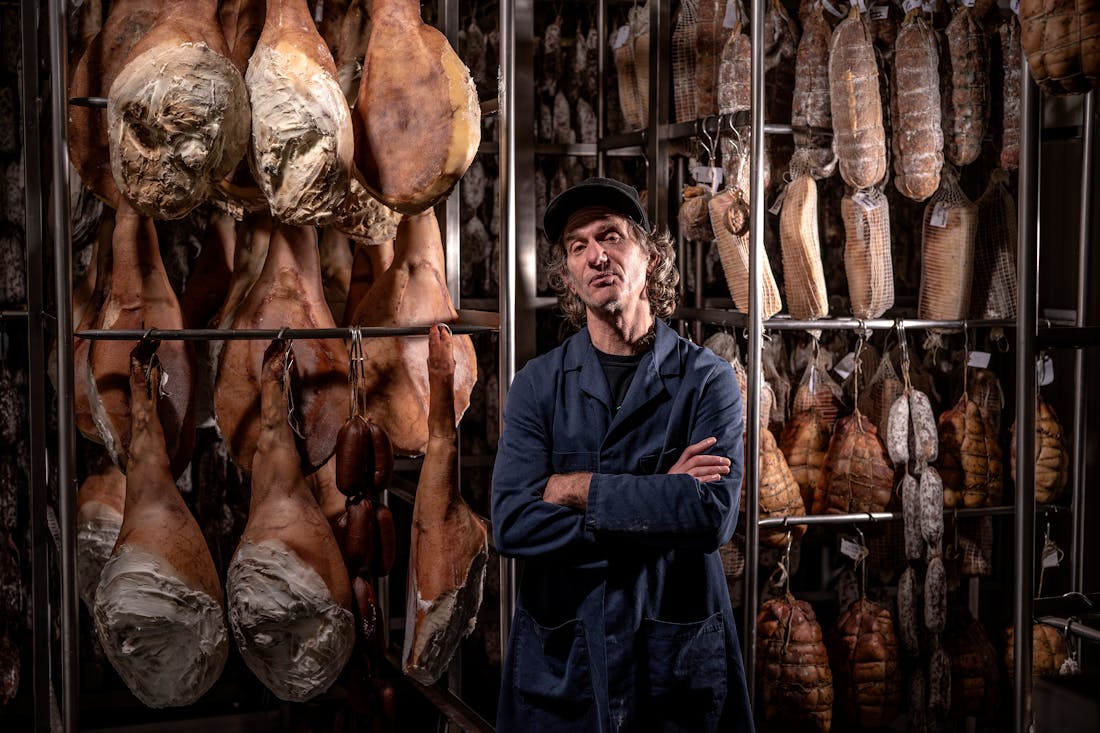In this image, a man stands at the center with his arms crossed, wearing a dark blue collared, long-sleeved button-down shirt over a darker undershirt, and a black cap over his curly brown hair. He gazes directly at the camera with a neutral expression. Behind him, the scene is filled with various meats hanging on stainless steel racks inside what appears to be a walk-in refrigerator or meat freezer. The meats, which include items resembling legs of lamb, turkey legs, salamis, and hams, are suspended on hooks from crossbars. These meats vary in appearance, with some wrapped in white cloth or cellophane and others plainly exposed. Despite the dim lighting, which casts darker shadows on the edges of the frame, the man and the hanging meats are clearly visible, filling the backdrop with an intricate display of preserved foods.